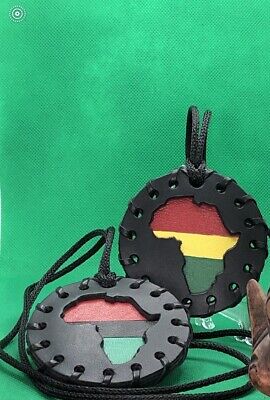The photograph features a close-up of two identical black circular leather medallion necklaces, each with a cutout in the shape of the African continent. Both necklaces are suspended by black ropes. The medallion on the left is positioned horizontally, displaying the African continent with red, black, and dark green stripes from top to bottom. The medallion on the right is oriented upright, revealing the continent with red, yellow, and green stripes from top to bottom. The background of the image is a dark green cloth, and there is an indistinct brown object visible along the right edge, possibly a glove. The overall size of the photograph is approximately two inches by three inches, and no further identifying information is provided.